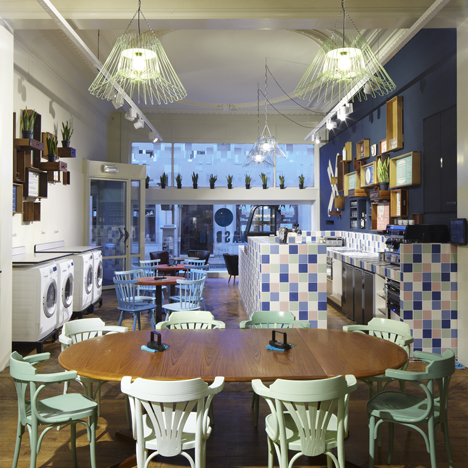In this image, we're inside a stylish, multifunctional kitchen and laundry room that could be part of a business establishment or restaurant. At the center, there's a light mahogany wooden table surrounded by eight seafoam green chairs and two blue items placed on top. The flooring is tiled, enhancing the room's clean and modern look. To the left, there's a row of four white washer and dryer units. The kitchen occupies the right side of the room, featuring deep sinks and ample shelving. The walls are mostly sky blue and adorned with framed pictures, shelves, and hanging plants, adding a touch of greenery. The ceiling is white with unique light fixtures, featuring exposed bulbs and white bars running across it. Near the glass-paneled front door, you can find more plants suspended from the ceiling. The overall color palette includes light mahogany, various shades of blue and green, white, black, and hints of pale pink, creating a vibrant yet cohesive atmosphere.